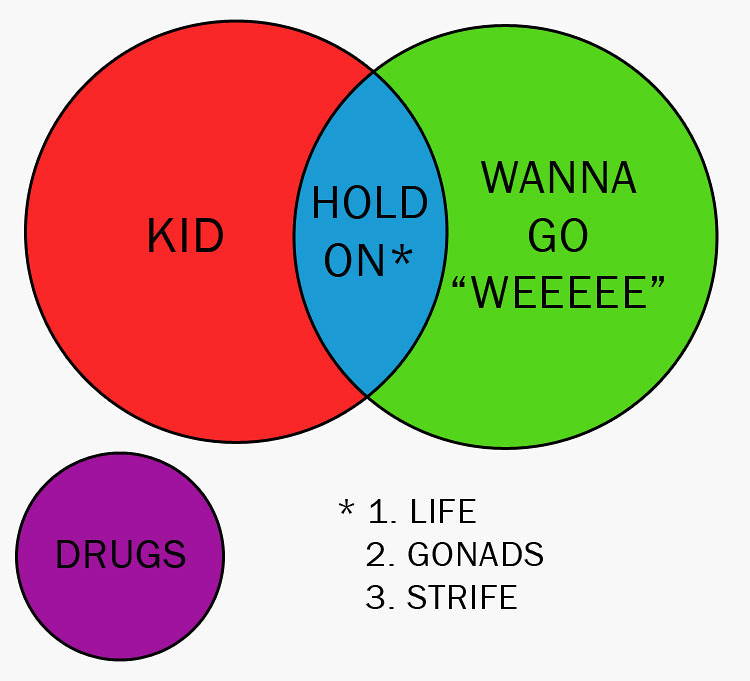The square-shaped image features a seemingly whimsical Venn diagram set against a solid white background. The diagram consists of three main circles: a large red circle labeled "kid" on the left, a large green circle labeled "wanna go 'weeeee'" on the right, and their overlap forms a blue section labeled "hold on" with an asterisk. Separately, in the bottom left corner, there’s a smaller purple circle labeled "drugs." Beneath the Venn diagram is a numbered list accompanied by an asterisk: 1. life, 2. gonads, 3. strife. The overall layout emphasizes a playful yet structured arrangement of concepts and elements.